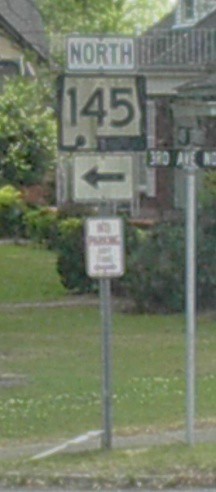In this vertically rectangular and narrow exterior image with natural low lighting, the slightly blurry background reveals a quaint front yard adorned with some shrubs in front of a home. Dominating the foreground are two traffic signs. To the right stands a shorter sign displaying a horizontal rectangular black sign with white lettering that reads "3rd Avenue." The left signpost is taller and features four different signs stacked vertically. At the top, a white sign with black lettering directs "North." Just below it, a larger square sign with a white background and black numbers reads "145." Beneath that, a smaller, slightly horizontally rectangular white sign displays a black arrow pointing left. At the very bottom, a small vertically rectangular white sign with red lettering warns "No Parking."